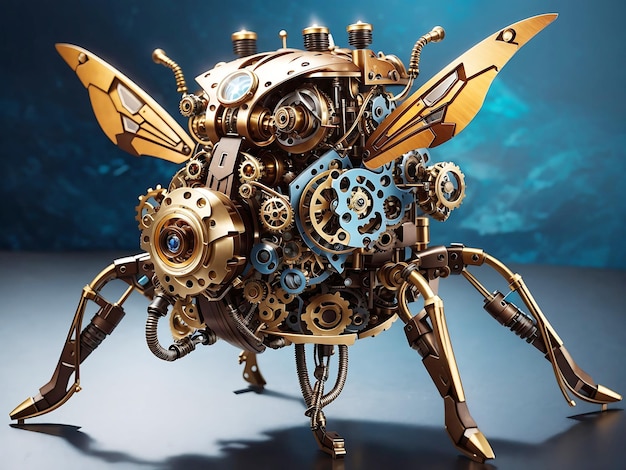This image features a highly detailed, mechanical insect-like creature that appears futuristic and animated. The creature’s body is constructed from various metallic gears, primarily gold with interspersed light blue elements. It stands on four gold, metallic legs, with an additional platform leg for support. The upper body comprises a series of gold and light blue wheels, giving it an intricate and open structure. Two small wings, colored yellow and brown, extend from its sides. The background transitions from dark blue on the left to light blue on the right, while the creature casts a shadow on a glossy light gray floor. The image is sharply zoomed in, emphasizing the intricacy and high quality of the mechanical design. The insect's head resembles a camera lens or drone-like feature, adding to its futuristic appearance.